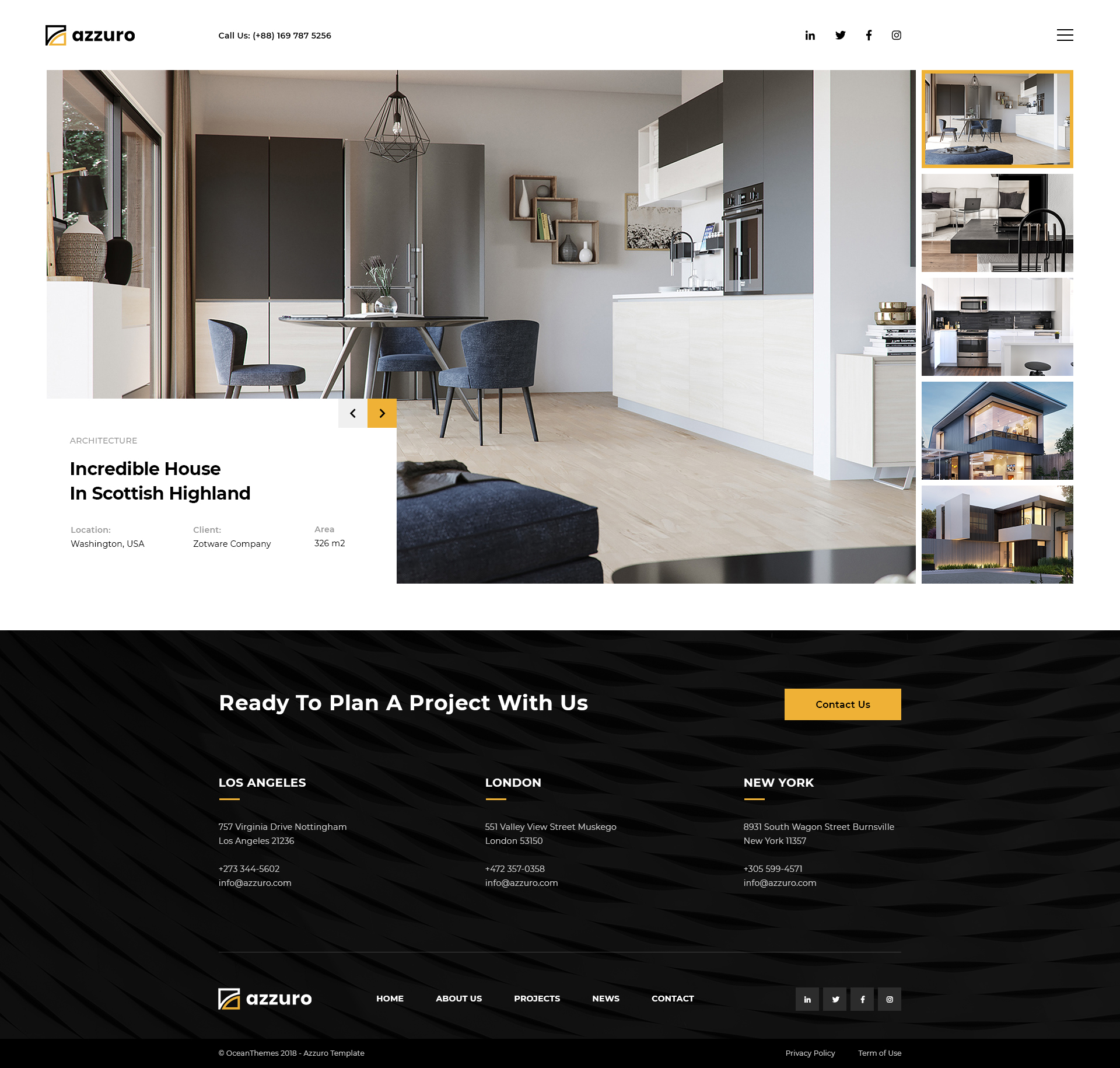This image showcases a detailed screenshot of a webpage, either from a tablet or a computer, representing a company named "Azuro." At the top of the page, the Azuro logo is prominently displayed, accompanied by a prompt to call them, although the phone number listed is difficult to read. The navigation bar includes icons for LinkedIn, Twitter, Facebook, and an unidentified icon resembling a cube, along with a menu symbolized by three horizontal bars.

Below this navigation bar, the main content area features a large image of a room, possibly a dining area or an eat-in kitchen, characterized by a round three-legged table surrounded by three blue padded chairs. Adjacent to the table is an easy chair, hinting at an open-plan layout that connects to a living room. The room is equipped with a white counter, cabinets, a high-placed oven, a possible sink at the far end, and distinctive décor including artwork and a small shelf displaying three flower pots. A notable feature is the elegant chandelier with a wrought iron grating encasing a single bulb. The refrigerator, a double-door model with distinct left and right sections, further complements the modern aesthetics of the room.

Beneath this primary image, there are five smaller thumbnails showcasing various views of the house. These include another angle of the kitchen with a black countertop and a black slatted seat, additional cabinetry which could suggest multiple kitchens or dining areas, and external views of a striking blue two-story house with a corner-wrapping big window. Another image displays the house from a broader perspective, revealing its predominantly white exterior and surrounding greenery.

Towards the bottom of the webpage, a prominent banner invites users to "Ready to plan a budget with us," accompanied by a yellow "Contact Us" button. Additionally, the page lists contact addresses and phone numbers for Azuro's offices in Los Angeles, London, and New York. The footer section includes navigation buttons labeled Home, Projects, and Contact, among other unreadable options.

This comprehensive caption provides a detailed overview of the webpage's content and layout, capturing the essence of both the interior and exterior features showcased.